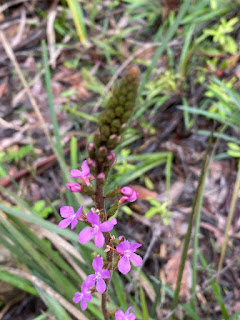The photograph captures a close-up view of a single plant in the wild, showcasing a vine with a green stem that rises just right of center from the bottom of the image, curving slightly to the left before extending upward. The top part of the stem deviates slightly to the right. The plant features small, fully bloomed purple flowers at the mid-section, their yellow centers adding contrast. Above these flowers, the stem thickens into a cylindrical green structure adorned with tiny green buds circling the top, which has a hint of brown at the tip. The background, depicted from an approximate 40-degree angle, reveals a patch of ground filled with grass, dirt, dry leaves, and weeds, adding earthy tones of brown and green to the scene. The environment suggests a small, grassy field, making the vibrant colors of the purple flowers and green stem stand out against the natural, muted backdrop.